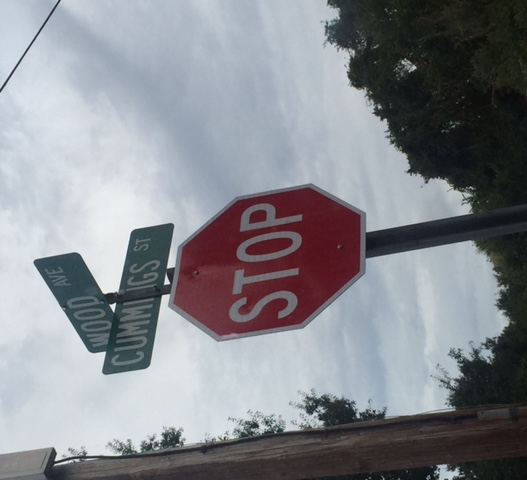In this photograph, we observe a busy intersection marked by street signs indicating Wood Avenue and Cummings Street, both mounted on a post that also holds a stop sign. The stop sign stands adjacent to an aged and weathered utility post. A wire stretches across the upper right corner of the frame, further adding to the scene's urban character. The sky is heavily overcast, blanketed in dense clouds that cast a gray hue over the entire area. Lush, older-growth trees form a dense tree line in the lower right corner and are also visible on the left side behind the utility post. This image captures the essence of a quiet intersection at Wood Avenue and Cummings Street on a cloudy, somber day.